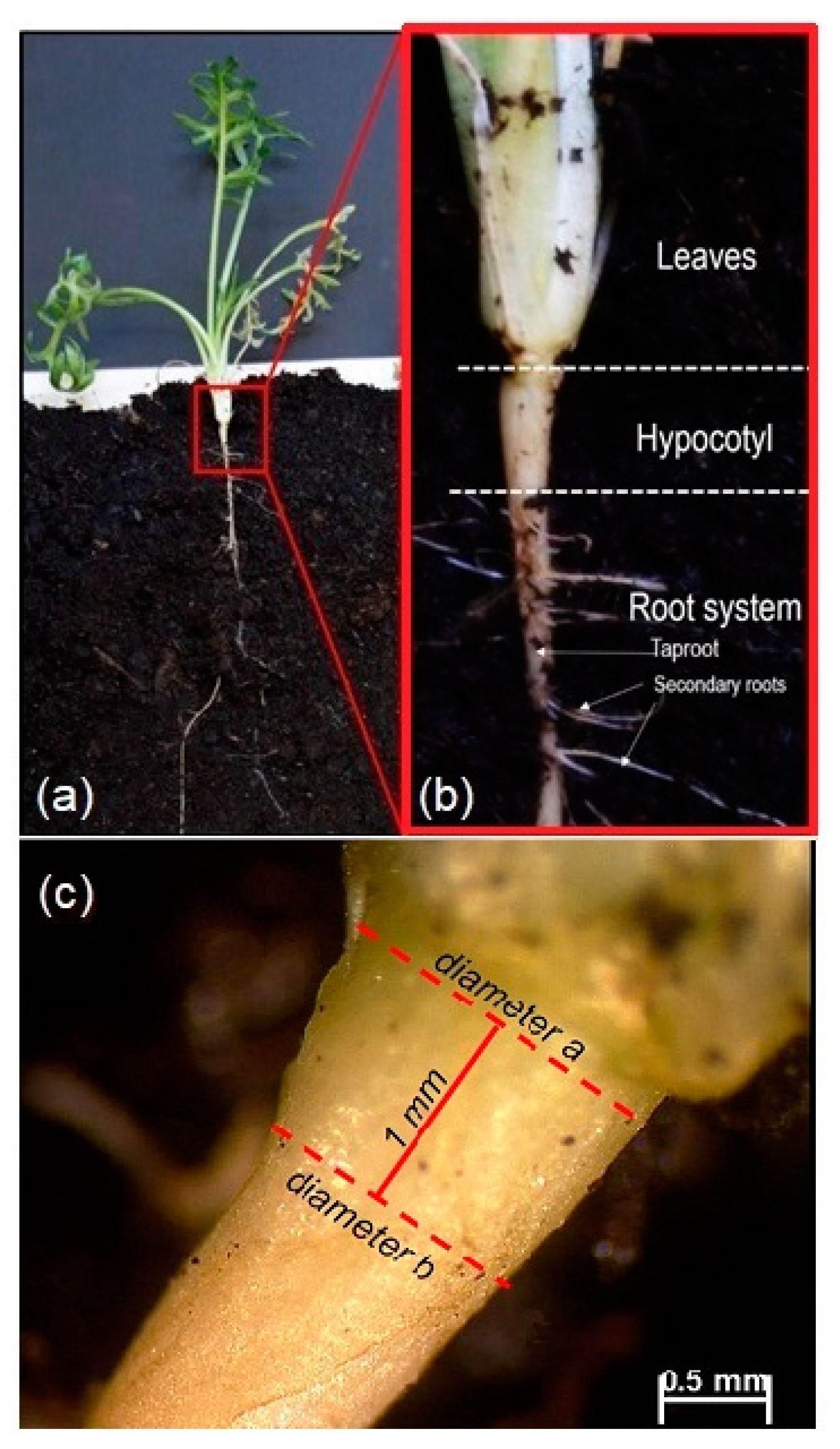The image is a vertically rectangular, full-color composition made up of three digitally enhanced photographs labeled A, B, and C. A displays a plant growing from dark brown soil, with green stems extending left and right. There's a red square around the root section, from which a red line leads to the C photo. Section B, marked by a red border, provides a zoomed-in view of the plant’s root system, highlighting key structural components such as the leaves, hypocotyl, tap root, and secondary roots. Dotted lines delineate these parts, with labels for each. C shows a detailed close-up of the tap root, colored light yellow, and includes red dotted lines and solid lines indicating diameters labeled as A and B, which are one millimeter apart. At the bottom of the image, there’s a measurement key showing a 0.5 millimeter segment to provide scale for the various sections.